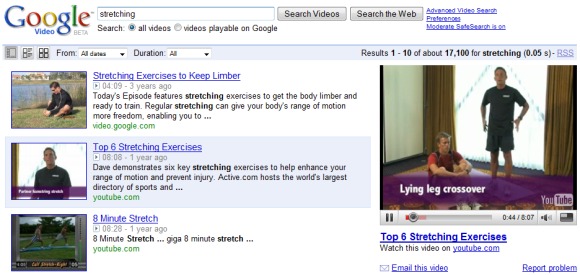The image features a screenshot of a Google search results page against a white background. The primary focus is on a Google search interface with a prominently placed search bar. Below the search bar are two gray rectangles labeled "Search Videos" and "Search the Web." 

The page includes three blue hyperlinks: "Advanced Video Search," "Preferences," and "Moderate Safe Search: On." Additional filtering options specify "From: All Dates" and "Duration: All." The search results show "Results 1 to 10 of about 17,100 for stretching," with the query completion time noted as "0.05s."

An RSS feed link is present, followed by three article headlines: "Stretching Exercises to Keep Limber," "Top Six Stretching Exercises," and "Eight-Minute Stretch." 

A featured video is paused at the 44-second mark of its total 8-minute and 7-second length. It is a YouTube video showcasing a woman seated on the floor stretching, with a man standing and also engaged in a stretching exercise. A red rectangle highlights this frame, including a white-lined leg crossover graphic. The video is titled "Top Six Stretching Exercises" with a prompt to "Watch this video on YouTube.com" in blue text.